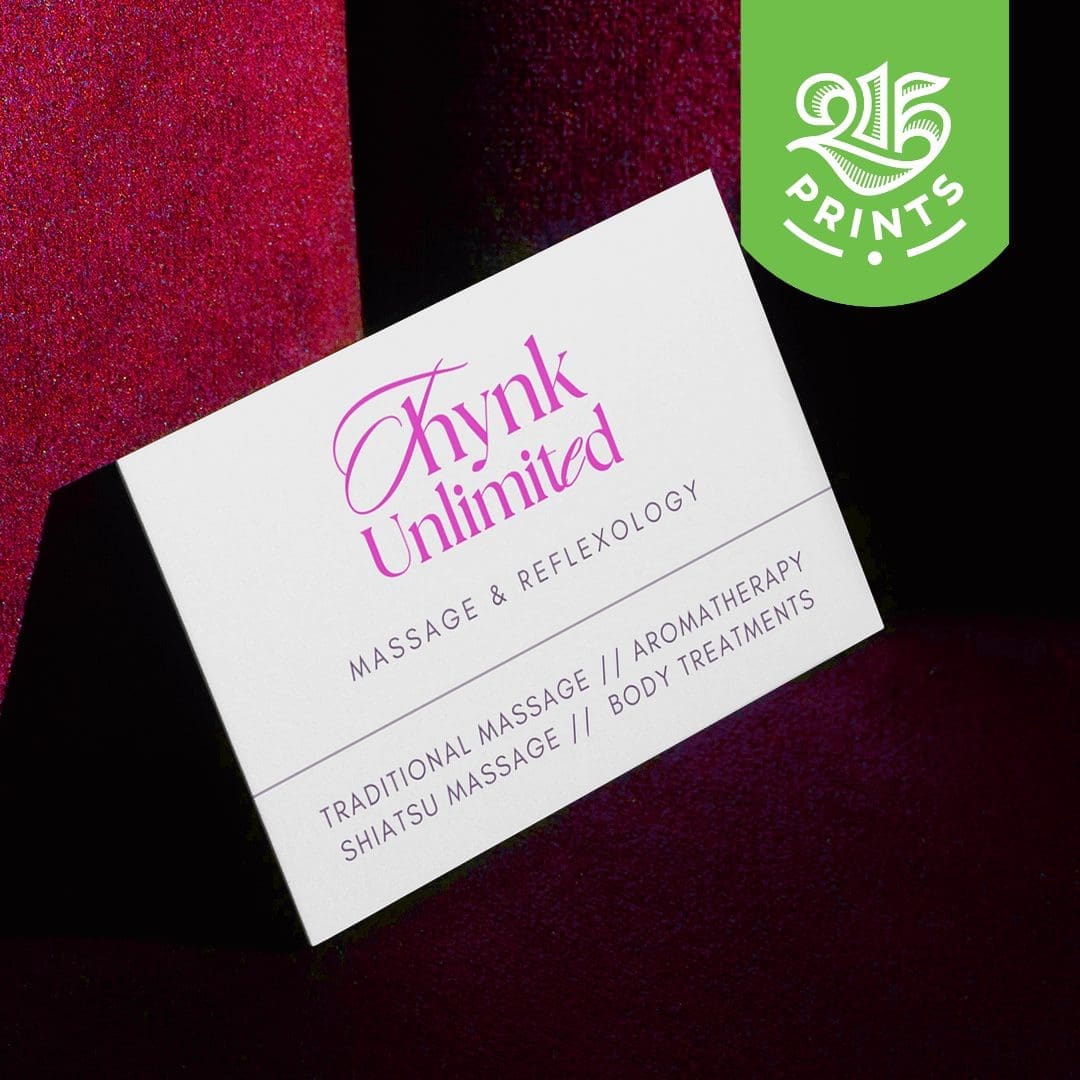This image showcases a mock-up of a business card promoting a massage and reflexology service by Think Unlimited. The business card features a white background with "THYNK UNLIMITED" in bright pink, the “T” is particularly stylized, and the “E” in “UNLIMITED” is italicized. Below that, in black text, it reads "Massage and Reflexology," followed by services listed in black: "Traditional Massage, Aromatherapy, Shiatsu Massage, Body Treatments." This card is set against a vibrant red, upholstered background resembling velvet, which variations in lighting give it a plush and dramatic appearance. In the top right corner of the image, on a green banner, is the logo "215 Prints," suggesting the card is an exhibit of their printing services. The business card is presented at an angle, enhancing its display appeal.